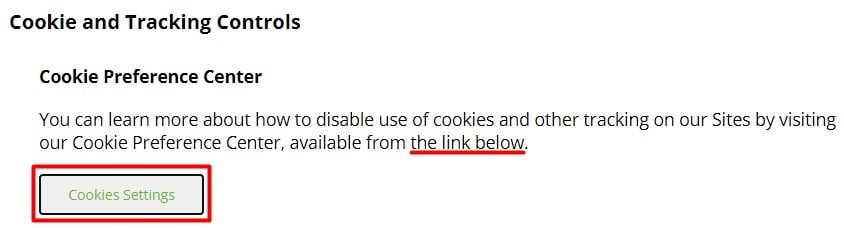The image features a detailed explanation of cookie and tracking controls on a website. At the top, bold black text reads "Cookie and Tracking Controls." Beneath this, an indented, smaller text states "Cookie Preference Center." Further text explains you can learn more about disabling cookies and other tracking mechanisms by visiting the Cookie Preference Center via a provided link. This link is underlined, signifying it is clickable, leading to further information or options.

Below this text, there is a gray button with a black border, containing green text that reads "Cookie Settings." A prominent red rectangle has been drawn around this button to emphasize the importance of clicking it to adjust your cookie settings.

This explanatory segment underscores the significance of managing cookie preferences, emphasizing that enabled cookies can personalize user experience by remembering site visits, but also highlighting privacy concerns due to potential tracking. Users are encouraged to carefully consider their cookie settings to balance convenience and privacy according to their preferences.